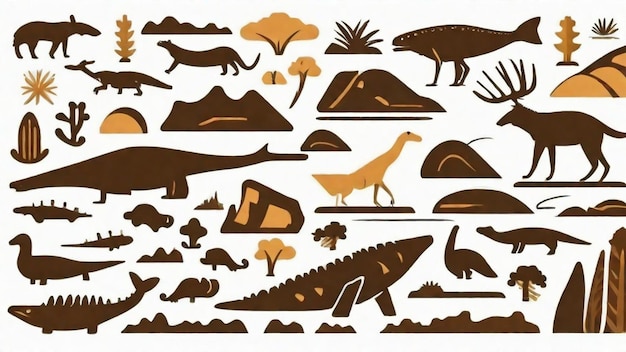The image is a rectangular artwork set against a white background, featuring a variety of minimalist animal and plant designs dominantly in brown and orange hues. The composition includes multiple creatures such as a brown, four-legged animal with a long-shaped nose situated at the top left. Adjacent to this creature is a brown-colored plant. Further to the right, there's a long-bodied animal with a pronounced tail. The array also includes fantastical and extinct animals like dinosaurs, a moose, and an imaginative fish with legs. The artwork is peppered with various types of plant life including trees, bushes, and cacti. The overall aesthetic resembles that of a kid's illustrated book, combining elements of whimsy and nature in a uniform color palette of two shades of brown.